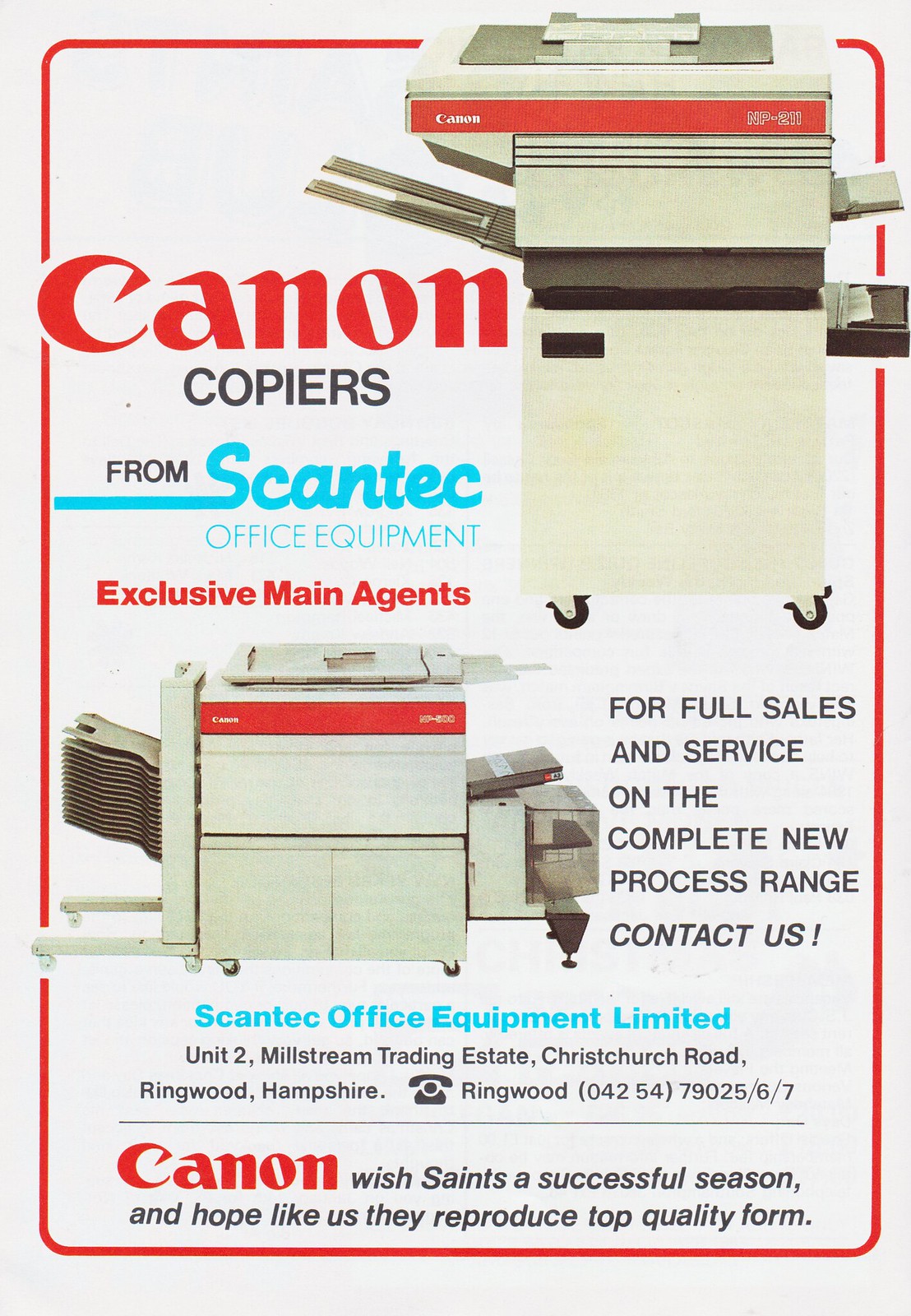This is a vertically oriented pamphlet advertising Canon copiers, prominently featuring the company's logo in red, with "copiers" in black text just below it. The upper portion showcases a photograph of a beige Canon copier with a distinctive orange stripe on top labeled "Canon." Adjacent text identifies that these copiers are available "from Scantech Office Equipment," the exclusive main agents for Canon. Further below, the pamphlet features another image of a Canon copier with a slightly different configuration, emphasizing the versatility and advanced capabilities of the product line. The advertisement highlights that Scantech Office Equipment provides comprehensive sales and services on the complete new range of Canon copiers. It lists detailed contact information: "Scantech Office Equipment Limited, Unit 2, Millstream Trading Estate, Christchurch Road, Ringwood, Hampshire, Ringwood 04254, 7902567," establishing the business's location in the UK.